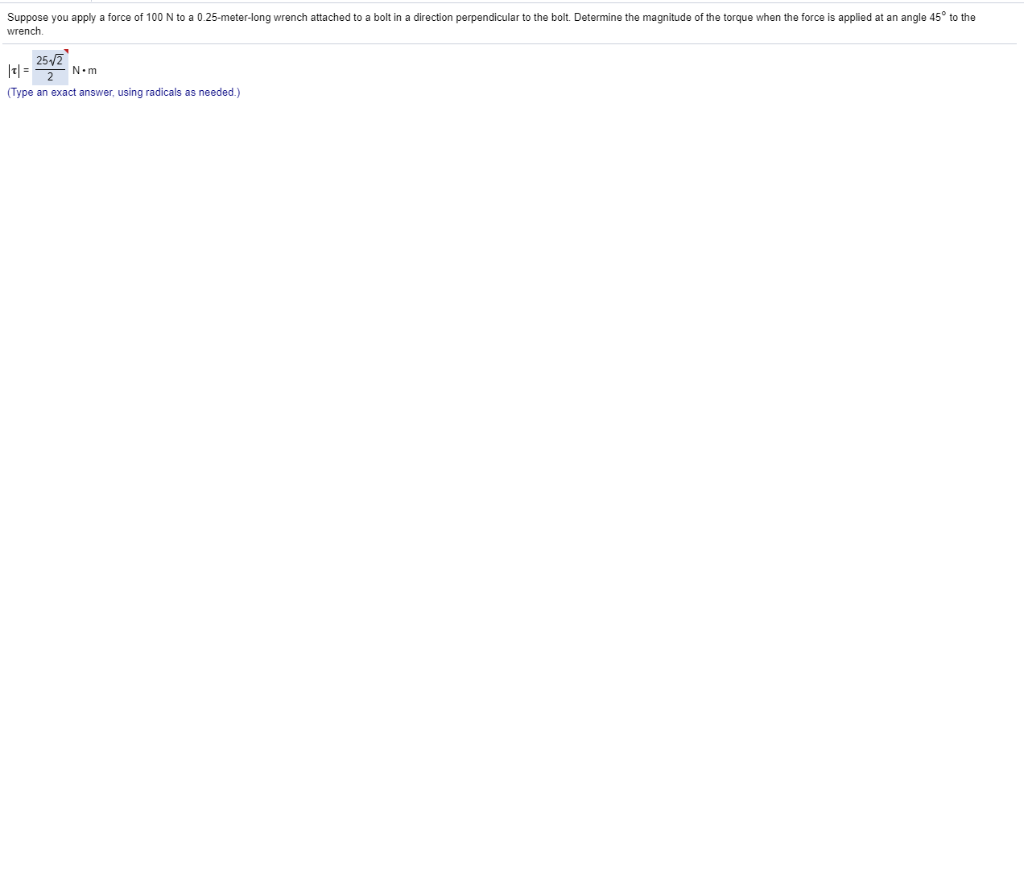In the image, we have a screenshot of digital text primarily set against a vast expanse of blank white space, occupying about 95% of the entire image. At the very top, there's a horizontal light blue line stretching from left to right. Below this line, black text is presented, reading: "Suppose you apply a force of 100 N to a 0.25 meter long wrench attached to a bolt in a direction perpendicular to the bolt. Determine the magnitude of the torque when the force is applied at an angle of 45 degrees to the wrench."

Following this text is a mathematical expression represented in digital typography. It consists of two vertical bars with a lowercase 'τ' (the Greek letter tau) inside them, possibly indicating torque. This is followed by an equal sign, leading into a light blue box that contains the value 25. Inside the box, there is a radical sign resembling a checkmark with a horizontal line extending from its top, containing the number 2. Underneath the radical sign is another number 2. To the right of this, outside the box, the text "Nm" (Newton-meters) is displayed.

In blue text beneath the equation, the instruction reads: "Type an exact answer using radicals as needed." This completes the detailed view and instructional content shown within the image.